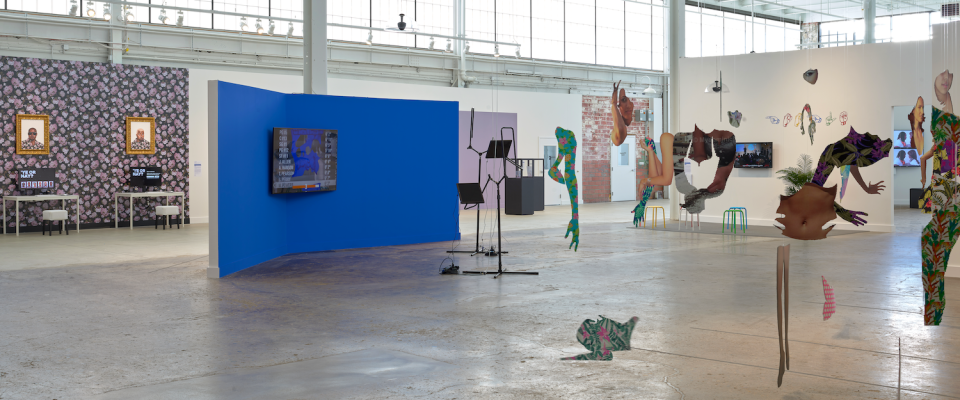The photograph depicts an expansive art museum housed within a warehouse-like space, characterized by its industrial aesthetic and open floor plan. The concrete floor and high windows allowing ample natural light set a stark stage for the eclectic array of artworks on display. Central to the scene is a prominent bright blue wall, featuring a large screen that could be a TV or incorporating 3D artwork, accompanied by conductor's stands in front. Suspended from the ceiling is a collection of unusual sculptures, which include pieces of animals, arms, and legs, creating an intriguing and somewhat fragmented visual theme.

To the left, a wall covered in dark blue wallpaper forms a backdrop to two white tables, each topped with a monitor and complemented by white stools. Above each table hangs an image of a person, enhancing the technological motif. The setup suggests a repeated theme throughout the museum, where TV screens dot various sections, situated on desks or against walls, possibly serving to explain the artworks or provide additional context. Continuing to the right, another section mirrors this layout, with additional white paneled walls, light fixtures, and televisions, framed by more stools. The entire space captures an intersection of modern technology and abstract art, creating an immersive and thought-provoking exhibit.